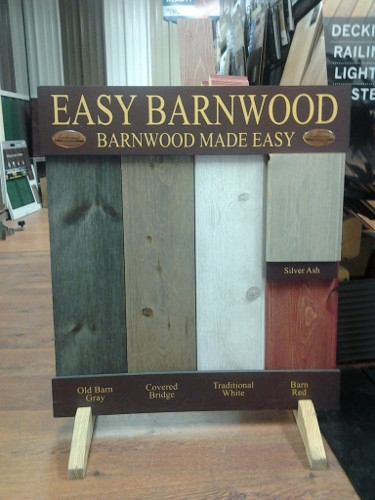This photograph captures an indoor store display of wood samples, illuminated by overhead fluorescent lights, indicative of an in-store setting. The display features a vertical rectangular signboard, standing on two light wooden legs placed on a hardwood floor. The top and bottom edges of the signboard are bordered with brown planks, with gold-lettered text reading "Easy Barnwood, Barnwood Made Easy" at the top.

The central portion of the display showcases five vertical wood samples in varying colors, each labeled with their corresponding names. From left to right, the samples are:

1. Old Barn Gray - a greenish-gray strip
2. Covered Bridge - a beige strip
3. Traditional White - a white strip
4. Silver Ash - a silvery gray strip 
5. Barn Red - a red strip with a small gray segment

Additional details include two small oval gold shapes with black text at the bottom corners of the sign, though the text is not legible. The background reveals more wooden panels hung from the ceiling and possibly some curtains, reinforcing the impression of a store interior. The top right corner of the image shows a partially cut-off sign.